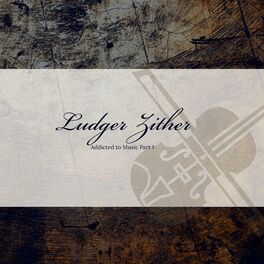The image displays an off-white business card placed on a marbled countertop or table. The right side of the business card features a clip art image of what seems to be a violin, complete with a bow crossing it. Even though it's unclear if the instrument might be a larger stringed instrument due to the scale of the image, the presence of the bow suggests it is most likely a violin. The text on the business card is slightly difficult to read due to the small size of the image, but it appears to say "Ludger Zither" in cursive script. Following that, there is an additional line of text reading "Addicted to Music Part 1," indicating possible involvement in music-related activities. It is assumed that Ludger Zither could either be offering violin lessons or is a violinist available for hire.